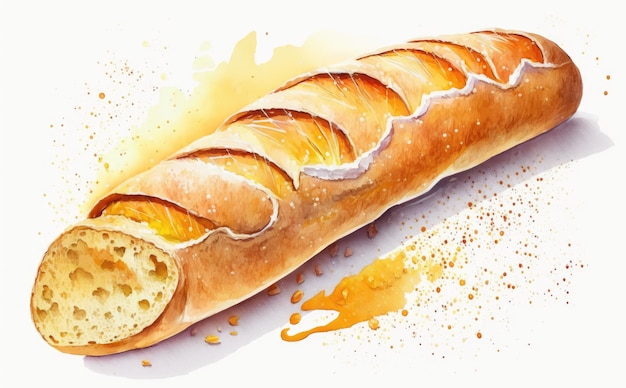This is a detailed watercolor illustration of a long, narrow French baguette. The bread is positioned diagonally from the bottom left corner to the top right corner of the painting, which has a plain white background. The artist has created a sense of texture and segmentation by painting notches along the top of the golden-brown baguette. Near the bottom left, the baguette is cut open, exposing a cross-section of its interior. Surrounding the bread and casting a light shadow beneath it, there are splatters of brown and orange watercolor, mimicking crumbs and seeds. These splatters, along with some yellow paint on the left side, add a dynamic and somewhat abstract element to the otherwise minimalist composition. The overall effect combines realistic details with a painterly style, giving the bread a semi-realistic, almost ethereal quality.